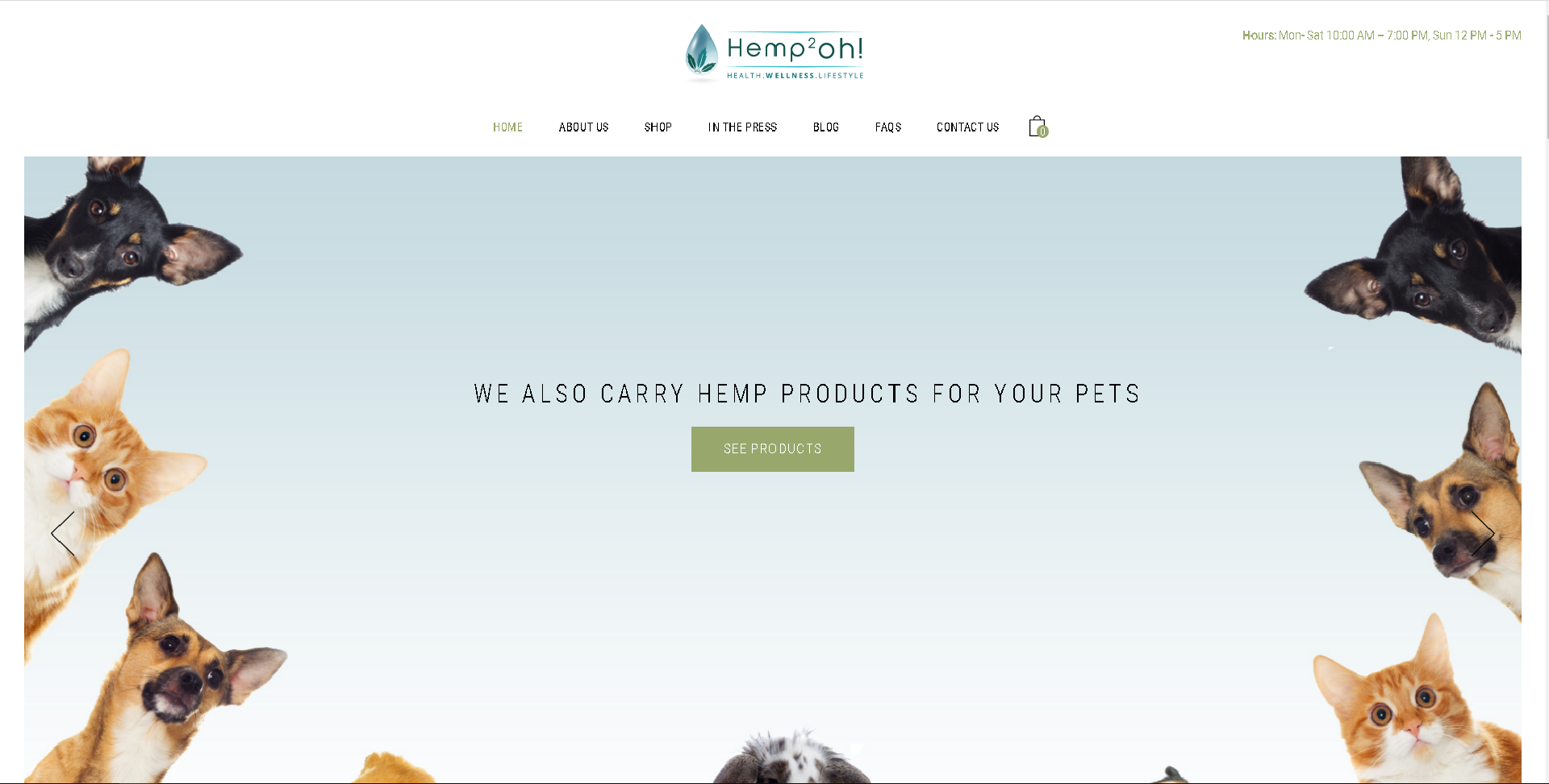Hemp Square-O's website homescreen features a predominantly blue and white background, creating a calm and inviting atmosphere for viewers. At the top of the page, the navigation menu includes options like "Home," "About Us," "Contact Us," "FAQ," "Blog," and "In the Press." 

In the center of the homepage, there is a prominent section labeled "See Products," which is highlighted in green with white text, drawing attention to the available products. This section is further enhanced by the tagline "We also carry hemp products for your pets" displayed in bold black text.

Around this central message, there are images of various pets, including cats and dogs. Specifically, there are depictions of six different animals, with a pattern alternating between cats and dogs. Another pet appears partially out of view, adding to the total count.

Overall, Hemp Square-O's homepage effectively communicates its focus on providing hemp products for pets through clear navigation and engaging visuals of cats and dogs.